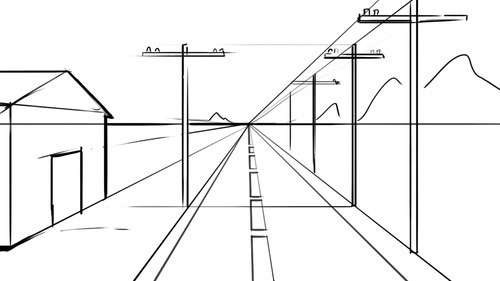A detailed black and white line drawing visually captures a stretch of a roadway leading toward a vanishing point on the horizon. The road, defined by parallel white lines on the edges and a dotted yellow line down the center, uses perspective to create a sense of depth as the lines converge at a V-shape on the horizon. On either side of the road, several tall telephone poles with wires stretching back emphasize the linear perspective. On the left side of the road, a simple, stick-figure-like drawing represents a five-sided house with a door and a roof marked by a horizontal line extending leftwards to imply a three-dimensional form. Contrasting the straightforward lines of the roadway and the building, the right side of the scene features curvy, wavy lines symbolizing hills or mountains rising in height as they approach the horizon. Above the horizon line, more horizontal and squiggly lines suggest clouds floating in the sky. The overall composition, primarily composed of straight and squiggly lines, illustrates a minimalist yet detailed expression of a highway scene meeting the horizon, with varied elements like buildings, telephone poles, and hills contributing to its simplistic yet vivid representation.